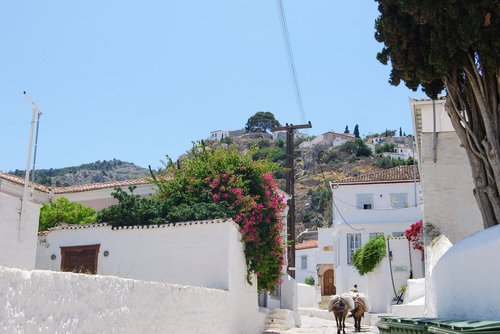This outdoor, rectangular landscape photograph captures a serene hillside village on a Grecian island. The scene includes a series of white, boxy stucco buildings with tiled roofs, some adorned with vibrant greenery and cascading shrubbery, and splashes of pink flowers. The village is nestled against a backdrop of rocky hills dotted with more white buildings. The sky above is a clear, light blue, indicating pleasant weather. A wooden telephone pole with wires runs vertically through the image, while a tall tree stands prominently on the right side, adding depth to the scene. Down the central path, slightly right off center, a man leads two laden donkeys away from the camera, further enhancing the rural and tranquil ambiance of this picturesque small town.